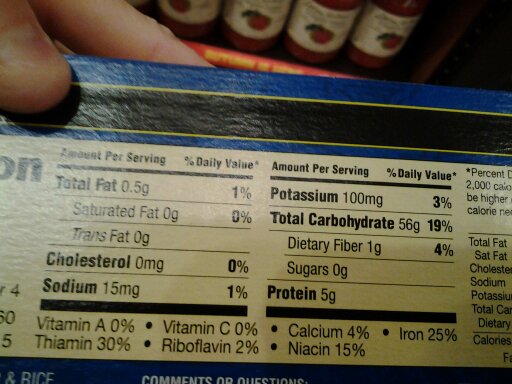A close-up image of the back of a food label is being held up by two fingers at the top. The label primarily shows the nutritional information of the food item, which remains unidentified. The nutrition facts listed include: total fat at 0.5 grams, saturated fat at 0 grams, trans fat at 0 grams, cholesterol at 0 milligrams, sodium at 15 milligrams, potassium at 100 milligrams, total carbohydrate at 56 grams, dietary fiber at 1 gram, sugars at 0 grams, and protein at 5 grams. At the bottom, additional nutritional details are presented: vitamin A at 0%, thiamin at 30%, vitamin C at 0%, riboflavin at 2%, calcium at 4%, iron at 25%, and niacin at 15%. The right side of the label continues with more text, which is not legible. The lower part of the label mentions "comments or questions." The background reveals three or four jars, possibly filled with salsa or spaghetti sauce, placed on a shelf or within a pantry.